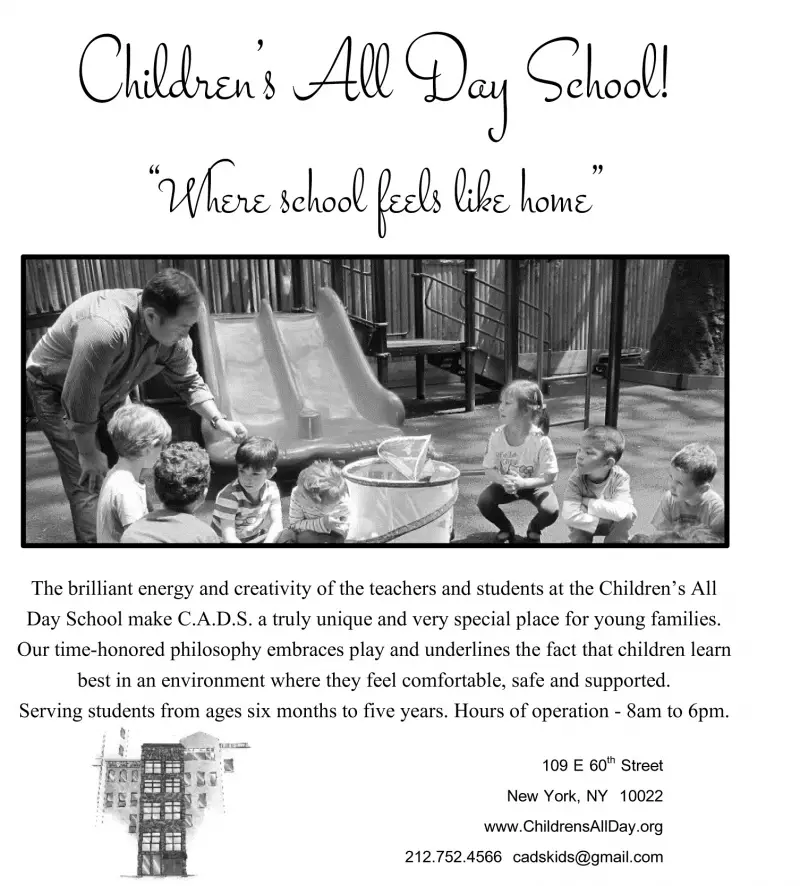The advertisement for the Children's All-Day School features a rectangular black-and-white photo at its center. In the photo, a man is leaning over and engaging with seven children, who are seated in a semi-circle around a bucket. This scene unfolds in a playground setting with visible slides and modern jungle gym equipment in the background. The man appears to be demonstrating something to the children, highlighting a moment of interactive learning. 

Above the photo, in cursive black text, the heading reads "Children's All-Day School," followed by the tagline in quotes, "Where school feels like home." Below the image, descriptive text emphasizes the school's unique and special environment, celebrating the brilliant energy and creativity of both teachers and students. It mentions the school's commitment to a play-based philosophy, stressing the importance of a safe and supportive environment for optimal learning. The school serves children from six months to five years and operates from 8 a.m. to 6 p.m.

Additionally, there is an illustrative image of a tall school building on the lower left corner, while the right side provides the school's address: "109 East 60th Street, New York, New York, 10022," as well as the website, "www.childrensallday.org," and contact information, "1-877-524-566-CADSKIDS@gmail.com."